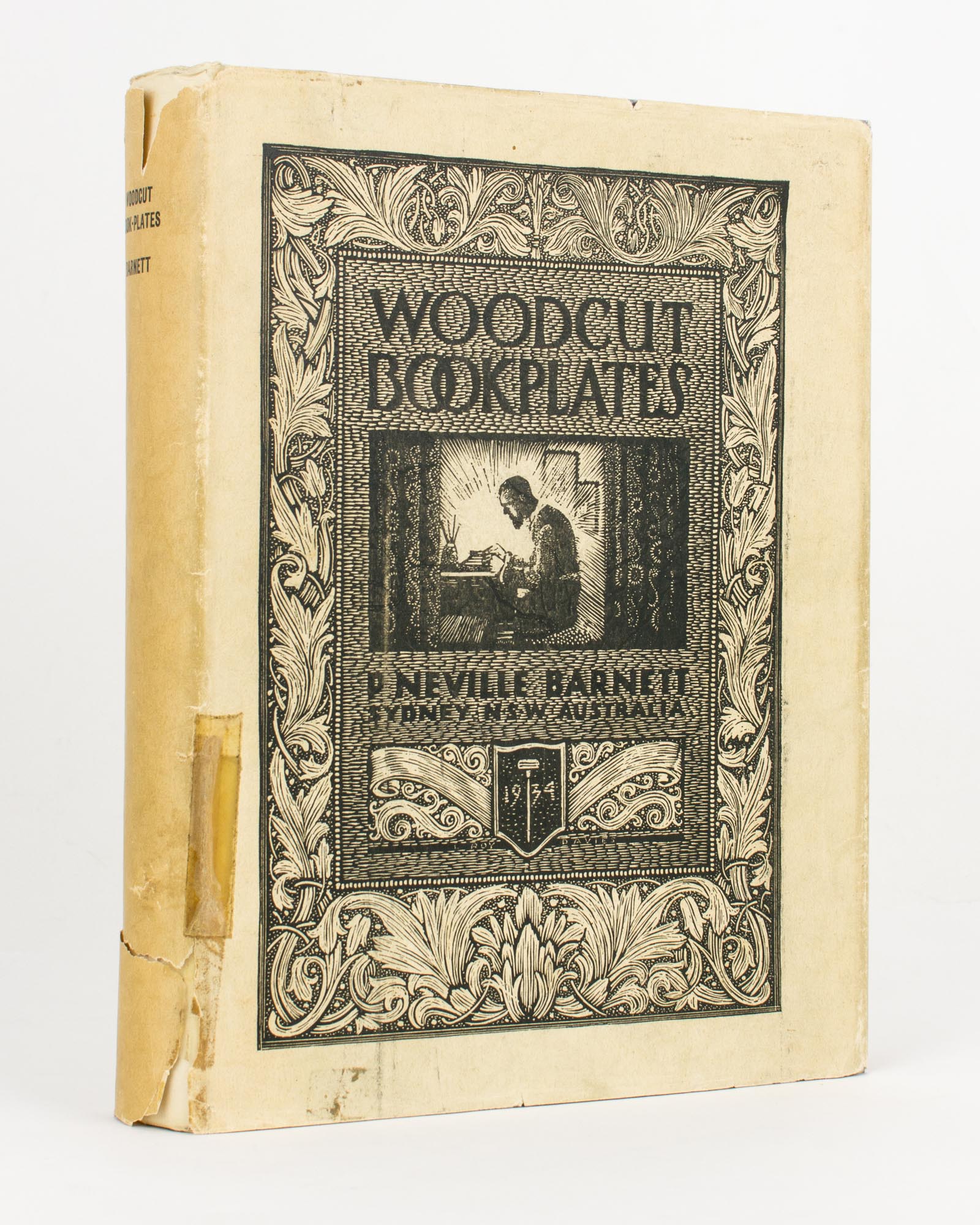The image features a vintage book titled "Woodcut Bookplates" by P. Neville Barnett, published in Sydney, NSW, Australia in 1939. The book, displayed vertically against a white background, shows significant signs of age and wear, with a faded cream-colored cover and a damaged spine held together with tape. The central focus of the cover is a detailed black ink illustration depicting a person working at a desk illuminated by a lamp, surrounded by books and papers. Above this illustration is the title "Woodcut Bookplates," and below, the author's name, P. Neville Barnett. The intricate design is framed by a decorative border of curved leaf patterns, enhancing the book's vintage charm and aesthetic. The overall scene evokes a nostalgic and elegant atmosphere.